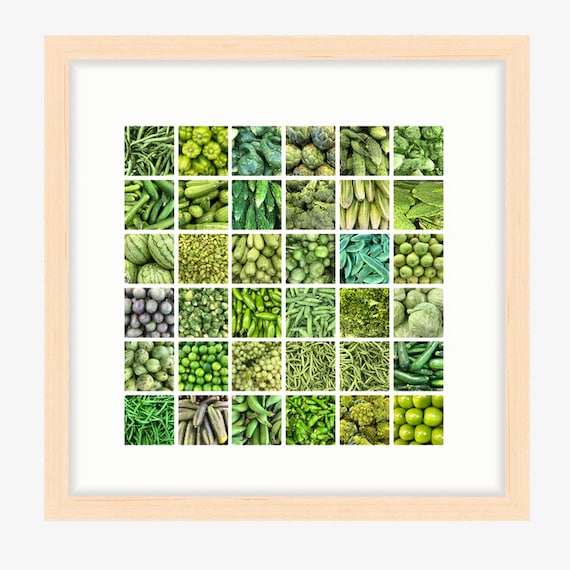This color photo, set in a peach-colored photo frame with a white background, features a detailed 6x6 grid collage showcasing a vibrant assortment of green-hued vegetation. Each of the 36 squares contains a close-up image of various fruits and vegetables, emphasizing the diversity in shades of green. Recognizable items within this verdant collection include peas, cucumbers, cabbage, watermelons, bell peppers, broccoli, artichokes, okra, green beans, Brussels sprouts, pickles, lettuce, and asparagus. Notably, one square diverges from the pervasive green palette with a hint of purple. The meticulous grouping of these plant images, devoid of any text, creates a visually captivating assembly of botanical variety.